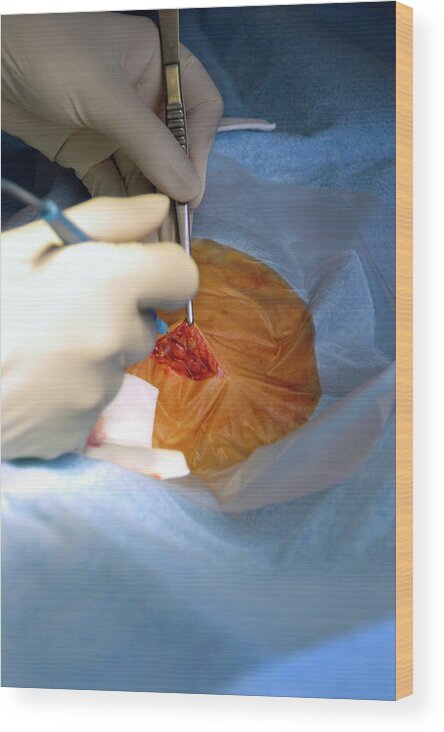The image, seemingly a traditionally styled photograph printed on canvas or wood, captures a close-up view of a surgical procedure. At the heart of the composition is the patient's open wound, encircled by a meticulously cut section of a light blue sterile gown. The doctor's hands, wearing white gloves, are engaged in the operation – one hand expertly wielding a silver scalpel and the other maneuvering a small blue power tool connected by a cable. The surgical scene, marked by the tan hue of the patient's skin and minimal bleeding, underscores the sterile and controlled environment of the hospital operating room. The arrangement places the wound centrally, with the gloved hands and surgical instruments positioned towards the top left, focusing the viewer's attention on the meticulous medical procedure.